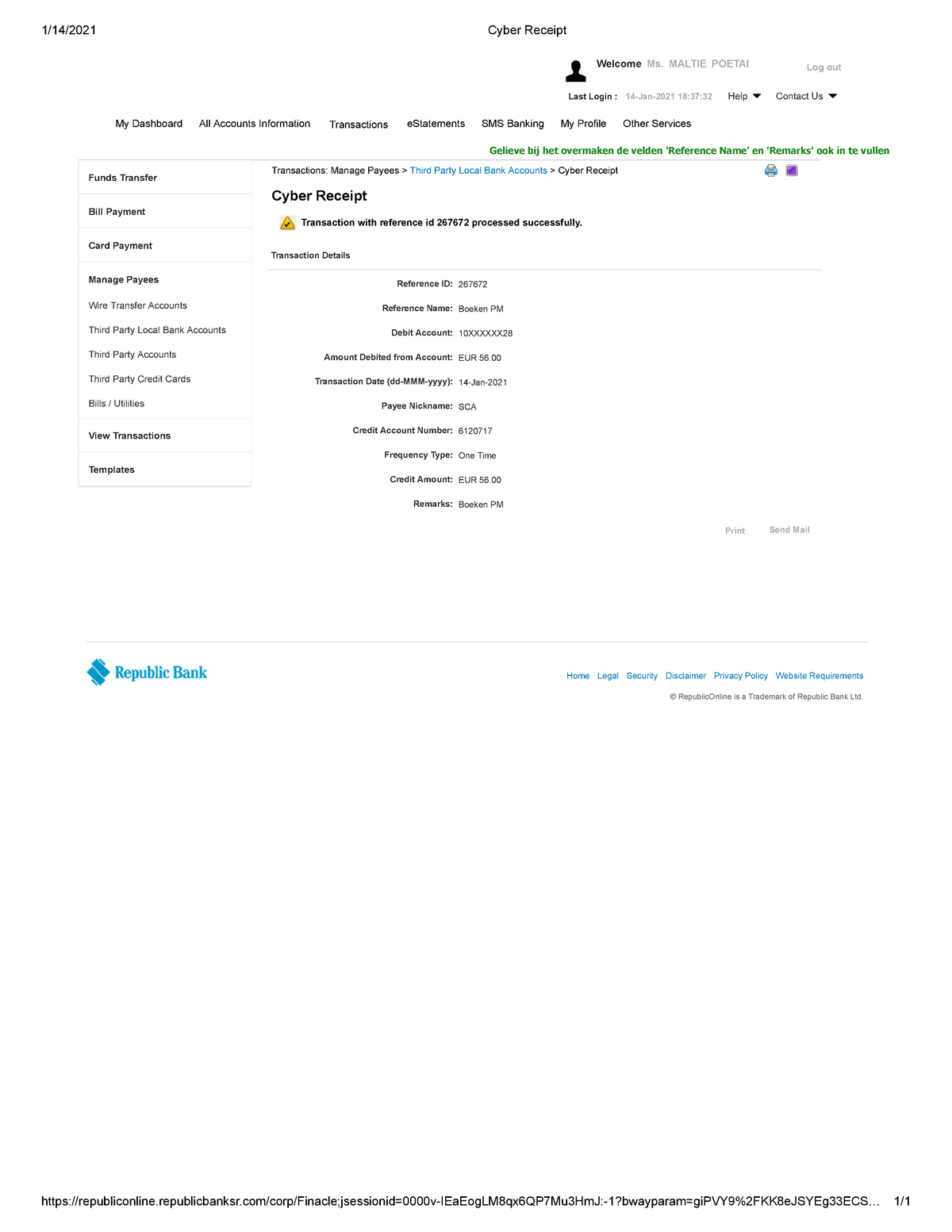On an all-white background, the image features a date, "01/14/2021," displayed in black in the top left corner. In the center, the text "Cyber Receipt" is written in black, with a small black icon of a human outline just below and slightly to the right of the "T". To the right of the icon, in bold black text, it says "Welcome." 

To the right of "Welcome," the text "Ms. Multi P O E T A I" is written in a dark grayish color, followed by a "Log Out" option. Below the image, the phrase "Last Log In" appears in black, accompanied by the date and time in gray to its right. Further right, the words "Help" and "Contact Us" are displayed in black, each with a drop-down tab.

On the left side, under the "Help" section, a vertical list in black text includes options like "My Dashboard," "All Accounts Information," "Transactions," "E-Statements," "SMS Banking," "My Profile," and "Other Services." The "SMS Banking" option is highlighted in green. Below this in green, the word "German" spans across the page to the right, and a black border frames the top and left side of the page.

This border encloses additional options such as "Fund Transfer," "Bill Payment," "Card Payment," and "Managed Payers," with six drop-downs under "Managed Payers." Adjacent to this, on the right side of the page, transaction details are listed under a bolded section titled "Cyber Report," followed by fields such as "Reference ID," "Reference Name," "Debit Account," and corresponding information.

In the bottom left corner, "Republic Bank" is written in blue next to the Republic Bank icon. On the right side, further information is provided, leaving a significant gap in the bottom half of the page where additional links and a clickable website in black letters are displayed across the bottom.